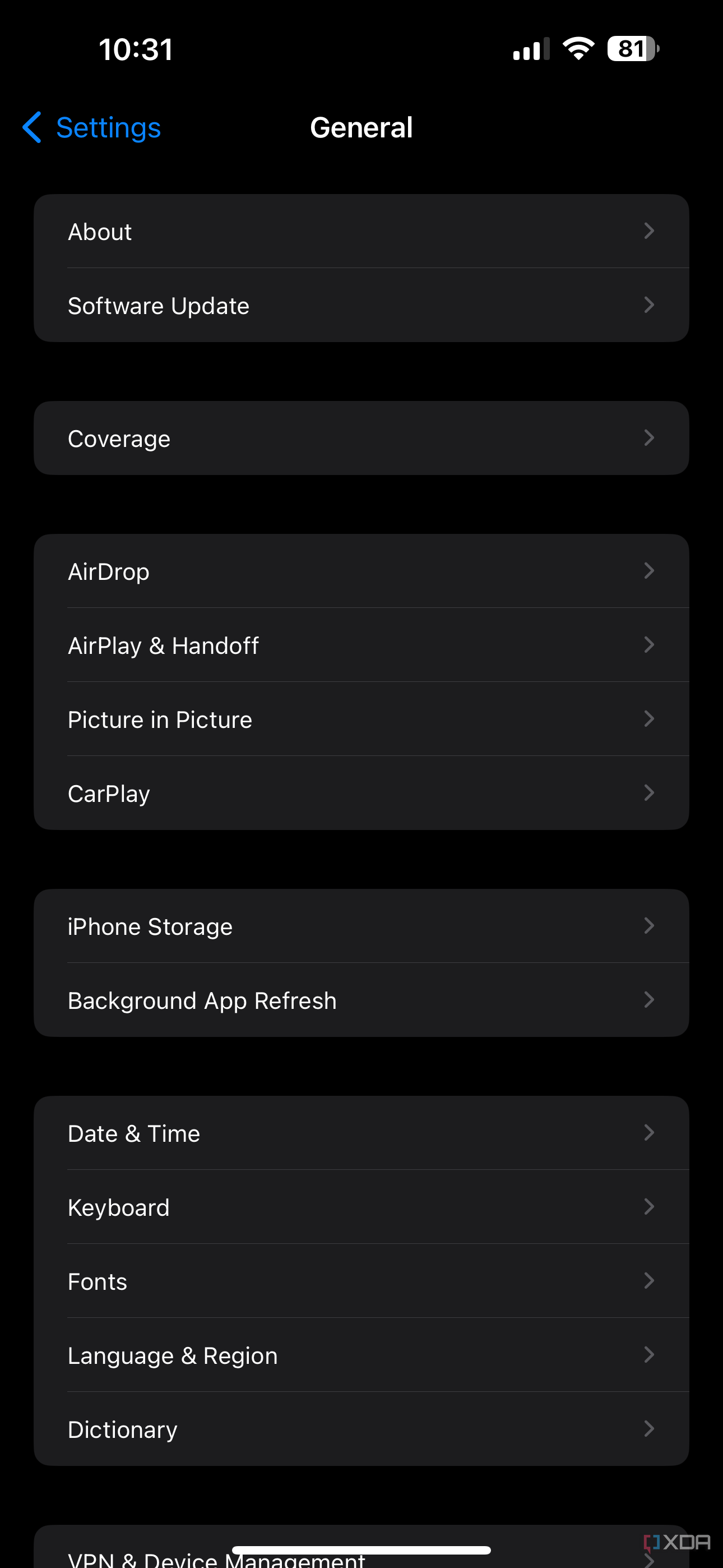A detailed screen capture of a smartphone displaying its settings menu, set in dark mode. The background features deep blacks and dark grays, enhancing readability. The status bar at the top shows the current time as 10:31, with strong signal strength and an 81% battery charge.

The settings menu is in the "General" tab, featuring several expandable options, each accompanied by an arrow indicating more information can be accessed. The "General" tab is organized into several groups of settings:

1. **First Group**:
   - **About**
   - **Software Update**

2. **Second Group**:
   - **Coverage**

3. **Third Group**:
   - **AirDrop**
   - **AirPlay & Handoff**
   - **Picture in Picture**
   - **CarPlay**

4. **Fourth Group**:
   - **iPhone Storage**
   - **Background App Refresh**

5. **Fifth Group**:
   - **Date & Time**
   - **Keyboard**
   - **Fonts**
   - **Language & Region**
   - **Dictionary**

At the bottom of the screen, partial text suggests additional options available via scrolling. The visible portion includes the "VPN & Device Management" option, indicating further settings below this point. This screen capture effectively demonstrates the detailed layout and organization of the phone's "General" settings menu.